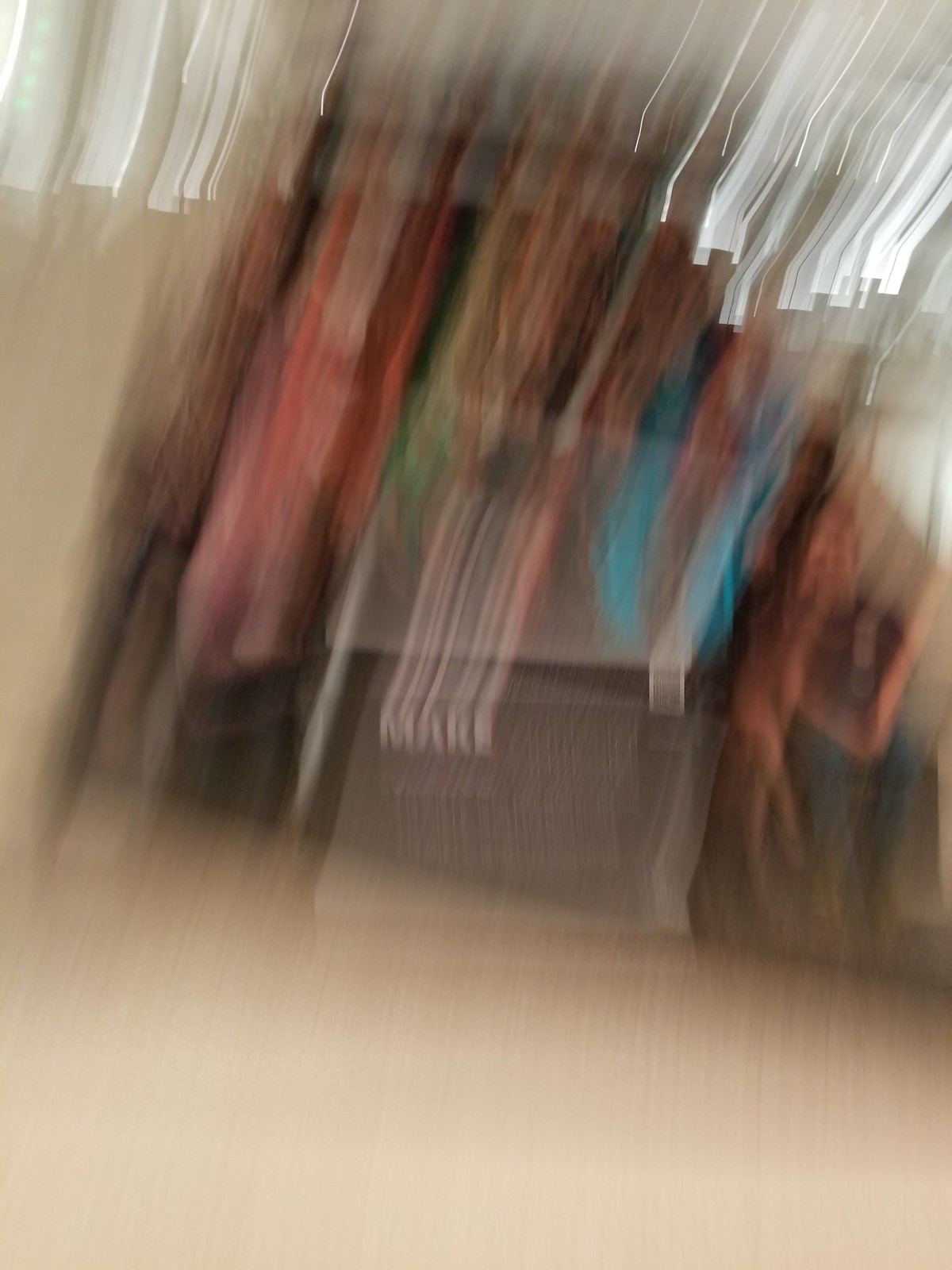In this highly blurry photograph, two figures are discernible on the left side of the image, sitting close together. The person closer to the camera appears to be dressed in jeans and a dark-colored short-sleeve shirt. The individual next to them seems to be sitting with crossed legs, but due to the blur and streaking effects, their details are difficult to make out clearly. 

On the right side, a colorful cardboard cutout catches the eye, displaying an array of hues including teal blue, red, white, gray, green, orange, and yellow. Below the colors, vaguely visible white lettering spells out "M-A-R-E." The surrounding environment includes what seems to be a white wall, a lighter-colored floor, and faint outlines of windows in the background, all adding to the indistinct atmosphere of the photo.